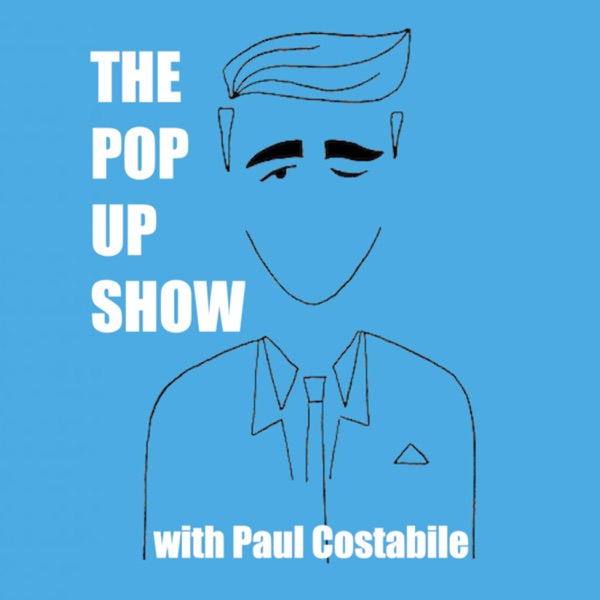The image is a blue-themed advertisement poster featuring white text and a stylized, low-detail sketch of a man. At the top left, in white letters, it reads "THE POP-UP SHOW," with each word stacked vertically. The center prominently displays the abstract outline of a man's head and upper torso, where only his hair, eyebrows, eye, sideburns, and jaw are clearly defined. He is wearing a suit with a tie and a handkerchief in the pocket, all depicted with minimal detail. The man appears to be winking; his right eye is open, while his left eye is closed. Below this illustration, the text reads "WITH PAUL KESTEMAEL" in white, located slightly above the bottom edge of the image. The color scheme of blue, white, and black emphasizes the minimalistic and almost abstract style of the poster, which serves as an advertisement for a show.